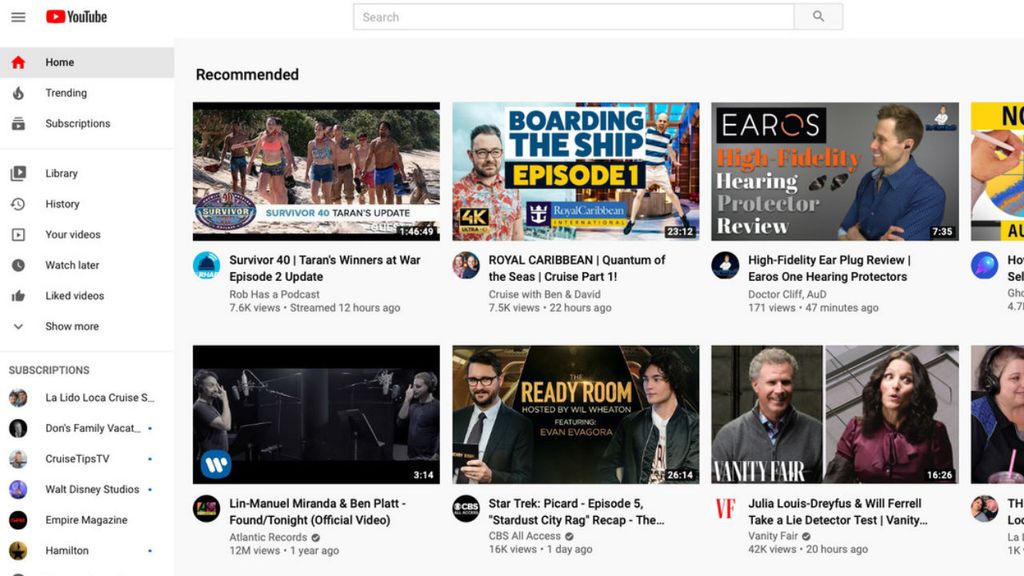This screenshot captures the interface of the YouTube homepage. It features a prominent, centrally located search bar at the top, which is currently empty but displays the word "Search". Below the search bar, various video thumbnails and links can be seen. These include a recap video of the Star Trek series, an earplug review, a clip from the TV series Survivor, and a music video titled "Found Tonight".

On the left side of the screen, a vertical menu provides navigation options. The menu includes the following links in descending order: Home, Trending, Subscriptions, Library, History, Your Videos, Watch Later, and Liked Videos. Near the bottom left corner, the interface lists the user’s subscribed channels, displaying their names.

The background of the webpage is entirely white. This detailed screenshot effectively shows key elements of the YouTube site layout.